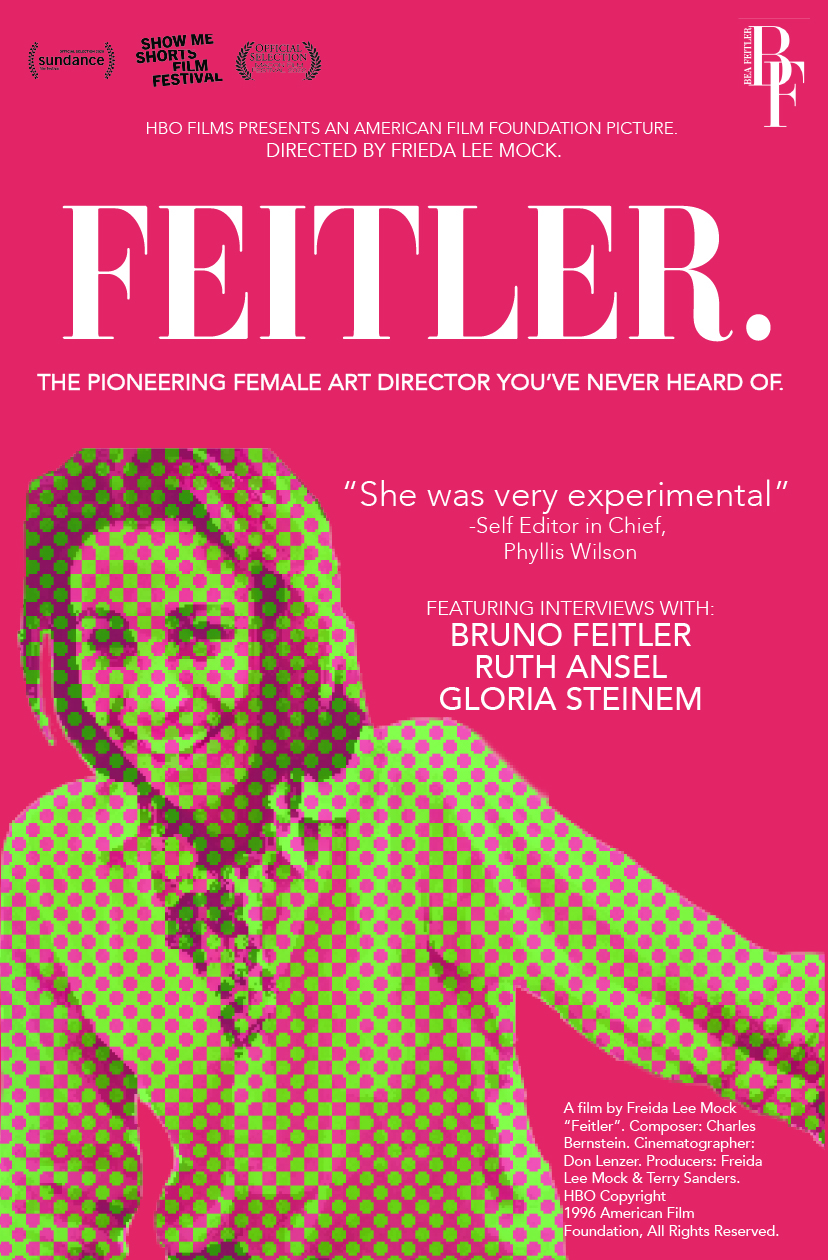The image is a red background movie poster for an HBO Films presentation by the American Film Foundation, directed by Frida Lee Mock. At the top, it lists accolades from the Sundance and Show Me Shorts Film Festival. The title "Feitler" is prominently displayed in bold, large white font. Beneath the title, the tagline reads, "The pioneering female art director you've never heard of." Below this is a quote, "She was very experimental," and it mentions Phyllis Wilson as editor-in-chief. The poster features an image of a young woman with brown hair, wearing a green shirt covered in pink polka dots, extending onto her face, creating a distinctive, distorted effect. The bottom right corner credits Frida Lee Mock as the director, and lists Charles Bernstein as the composer and Don Lenzer as the cinematographer. The poster also highlights interviews with Bruno Feitler, Ruth Ansel, and Gloria Steinem.